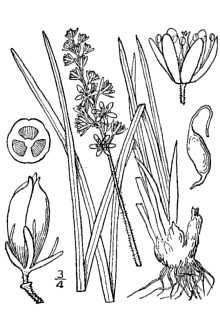This is a meticulous black and white hand-drawn image illustrating various parts of different plants. On the right side, the drawings depict the intricate root systems and blade-like leaves extending upwards. Central to the image is a plant stem adorned with multiple small flowers, showcasing both opened and closed blossoms. The upper sections highlight detailed views of the flowers, including a fully opened bloom and a closed bud. On the bottom left, there’s a detailed depiction of a flower bud nearing the point of opening, along with a cross-section revealing three equidistant internal pods. Close by, graphics of flower bulbs and a comprehensive root system extracted from the soil enrich the botanical detailing. The image captures the essence of plant anatomy, spanning from seed and root to full bloom, all in precise outline sketches.